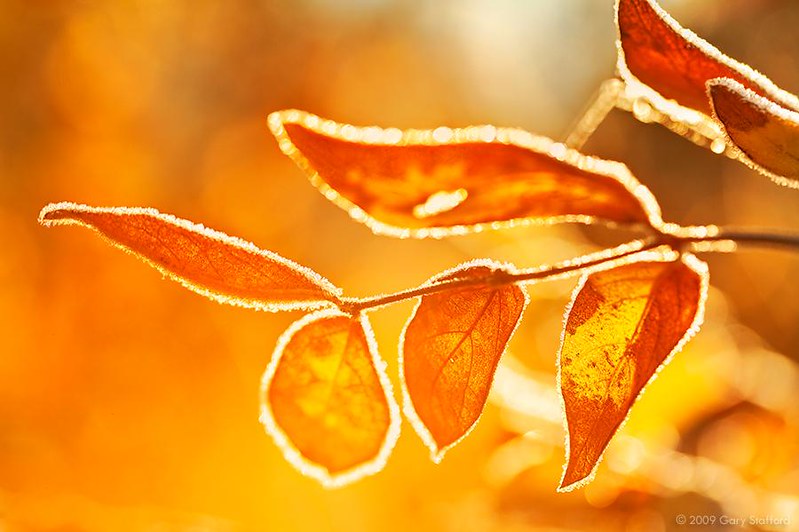A captivating close-up of a thin branch adorned with several small leaves, all immersed in an intense orange and yellow glow. The branch enters the frame from the right, extending about two-thirds towards the left, with three tiny leaves neatly spaced on either side. The overall scene is bathed in a warm, golden, almost amber hue, suggesting the use of a yellow filter that transforms the natural colors to appear bright orange. The background transitions smoothly from darker to lighter shades of orange, creating a gradient that emphasizes the vibrant tones of the leaves. Radiating from behind, the sunlight creates a striking halo effect around each leaf, which is delicately rimmed with frost, indicating an early morning frost that has lightly touched the plant. The background is artistically blurred, making the sharply focused leaves and their frosted edges stand out prominently against the soft orange backdrop. This photograph, taken in 2009 by a photographer named Gary, captures the ethereal beauty of a frosty, sunlit morning.